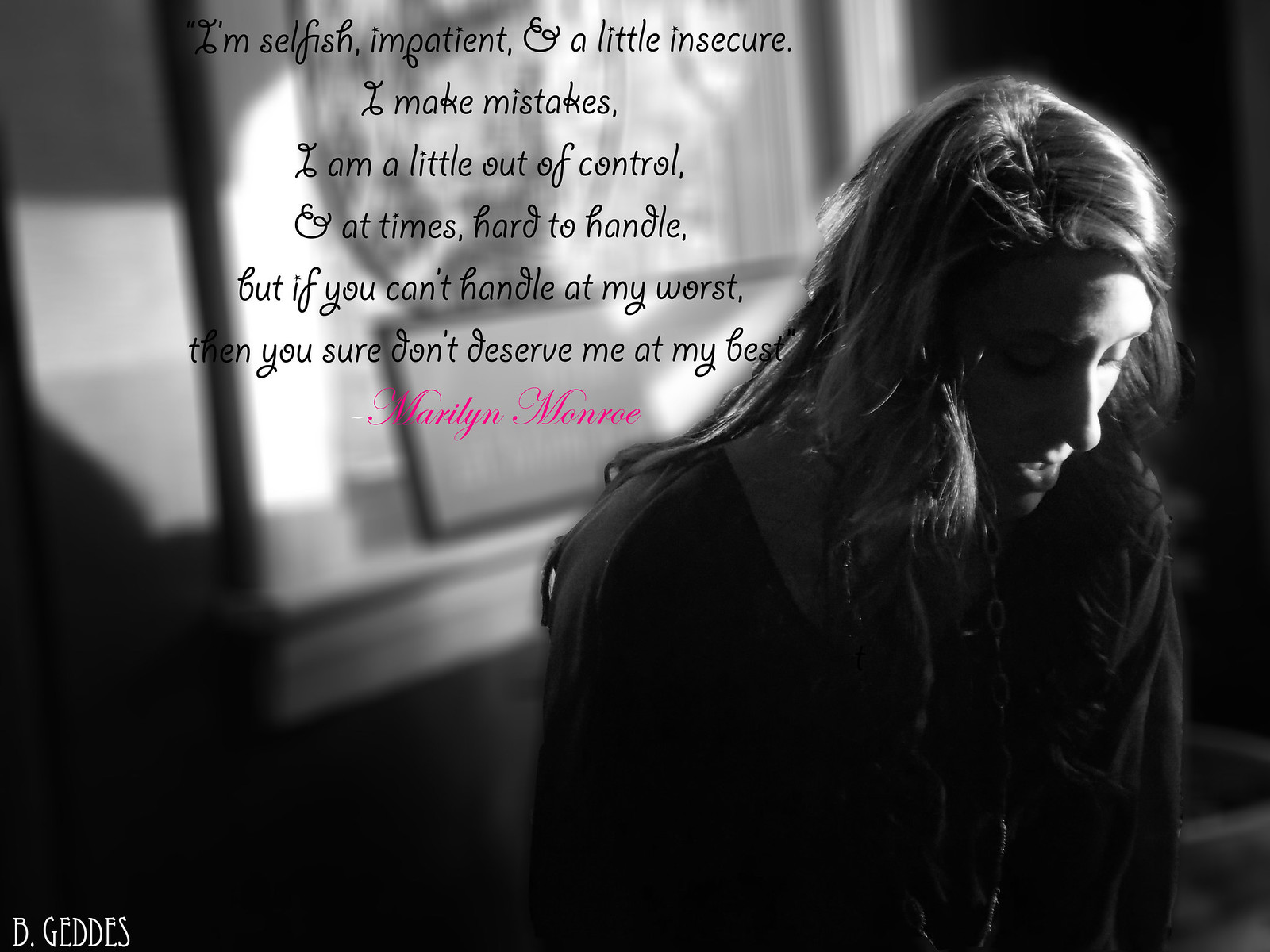The black and white photograph features a woman with long, likely blonde hair, positioned on the right side of the image and looking down. Her attire includes a jacket. Beside her on the left side of the photograph, there is a poignant quote written in black text: "I'm selfish, impatient, and a little insecure. I make mistakes, I am a little out of control, and at times hard to handle. But if you can't handle me at my worst, then you don't deserve me at my best." Below this quote is the name "Marilyn Monroe" inscribed in a hot pink, cursive italicized font. In the bottom right corner of the image, the name "B .GEDDES" appears in blue uppercase letters. The background is blurry but seems to depict either a window or a piece of art hanging on a wall.